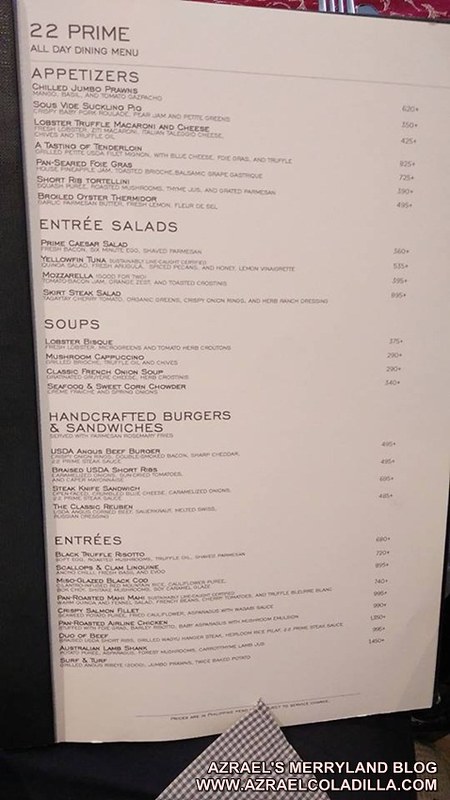This detailed photograph captures a comprehensive look at a restaurant's menu, prominently featuring the logo and URL "Azriel's Maryland Blog" (www.azrielpolita.com) in white letters at the bottom right. The menu has a clean white background, with "22 Prime All-Day Dining Menu" printed at the top left corner. 

The menu starts with a section on appetizers including:
- Chilled Jumbo Prawns
- Sous Vide Suckling Pig
- Lobster Truffle Macaroni and Cheese
- A Tasting of Tenderloin
- Hand-Seared Foie Gras
- Short Rib Tortellini
- Broiled Oyster Thermidor

Following the appetizers, the entree salads listed are:
- Prime Caesar Salad
- Yellowfin Tuna
- Mozzarella Salad
- Skirt Steak Salad

The soups section includes:
- Lobster Bisque
- Mushroom Carpaccio
- Classic French Onion Soup
- Seafood and Sweet Corn Chowder

Next, the menu presents a selection of handcrafted burgers and sandwiches:
- USDA Angus Beef Burger
- Braised USDA Short Ribs Sandwich
- Steak Sandwich
- The Classic Reuben

The entrees feature a variety of dishes such as:
- Black Truffle Risotto
- Scallops and Clam Linguine
- Miso-Glazed Black Cod
- Pan-Seared Mahi-Mahi
- Crispy Salmon Fillet
- Pan-Roasted Chicken
- Duo of Beef
- Lamb
- Surf and Turf

With this detailed lineup, the restaurant promises a culinary experience fit for any dining occasion.